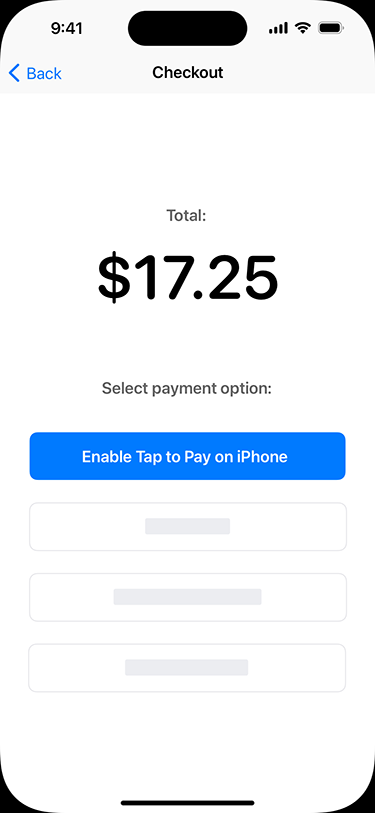The image depicts a smartphone screen displaying a payment interface. At the top of the screen, the current time is shown as 9:41, accompanied by standard status indicators for signal strength, Wi-Fi, and battery percentage. Prominently centered beneath the status bar is a cutout for the front-facing camera.

Below this, the screen features a blue back button on the upper left, followed by bold black text reading "Check Out" in the center. The total amount due is clearly listed as $17.25. Directly underneath, gray text instructs the user to "Select Payment Option."

A prominent blue icon, located further down, prompts the user to "Enable Tap to Pay on iPhone." Surrounding this are three additional boxes for other payment options, though they are currently grayed out, indicating that they are not selectable at this moment.

The lower portion of the screen includes a black navigation bar centered at the bottom, with black quarter circles on either side, against an overall white background. The interface is clean and minimalistic, featuring various text boxes and blue buttons to facilitate user interaction.

This appears to be a screenshot of a digital payment screen, likely to be used for in-store purchases via a mobile device, highlighting the option to tap and pay at a merchant's checkout.